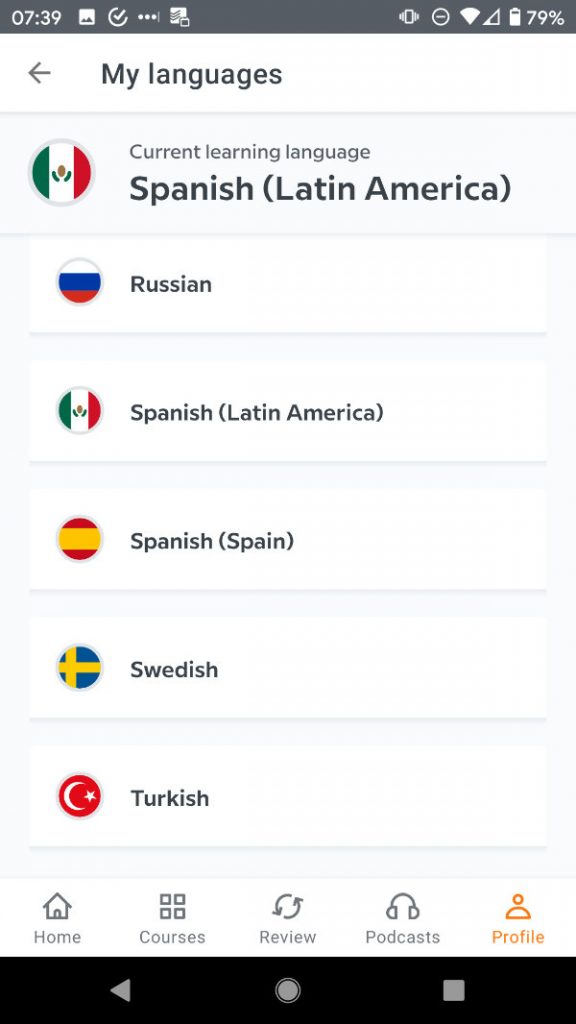The image is a screenshot of a language learning mobile application interface. At the top, the standard mobile status bar is visible with a grey background. The time displayed is 7:39. To the right of the time, four icons are present: the Wi-Fi icon, and the battery icon indicating a 79% charge.

Directly below the status bar, the header area shows "My Languages," accompanied by a back button on the left-hand side. A thin grey line separates the header from the rest of the interface.

The main content area contains a list of language options, each represented with a button. The currently selected learning language is "Spanish (Latin America)." Following options are listed in order: "Russian," "Spanish (Latin America)" again, "Spanish (Spain)," "Swedish," and "Turkish."

At the bottom of the screen, there is a navigation bar with five icons: Home, Courses, Review, Podcasts, and Profile. The Profile icon is highlighted in orange, indicating it is the currently selected section.

Below this navigation bar, there is a black rectangular box with three icons, suggesting media controls: a rewind or back button on the left, a record button in the center, and a stop button on the right.